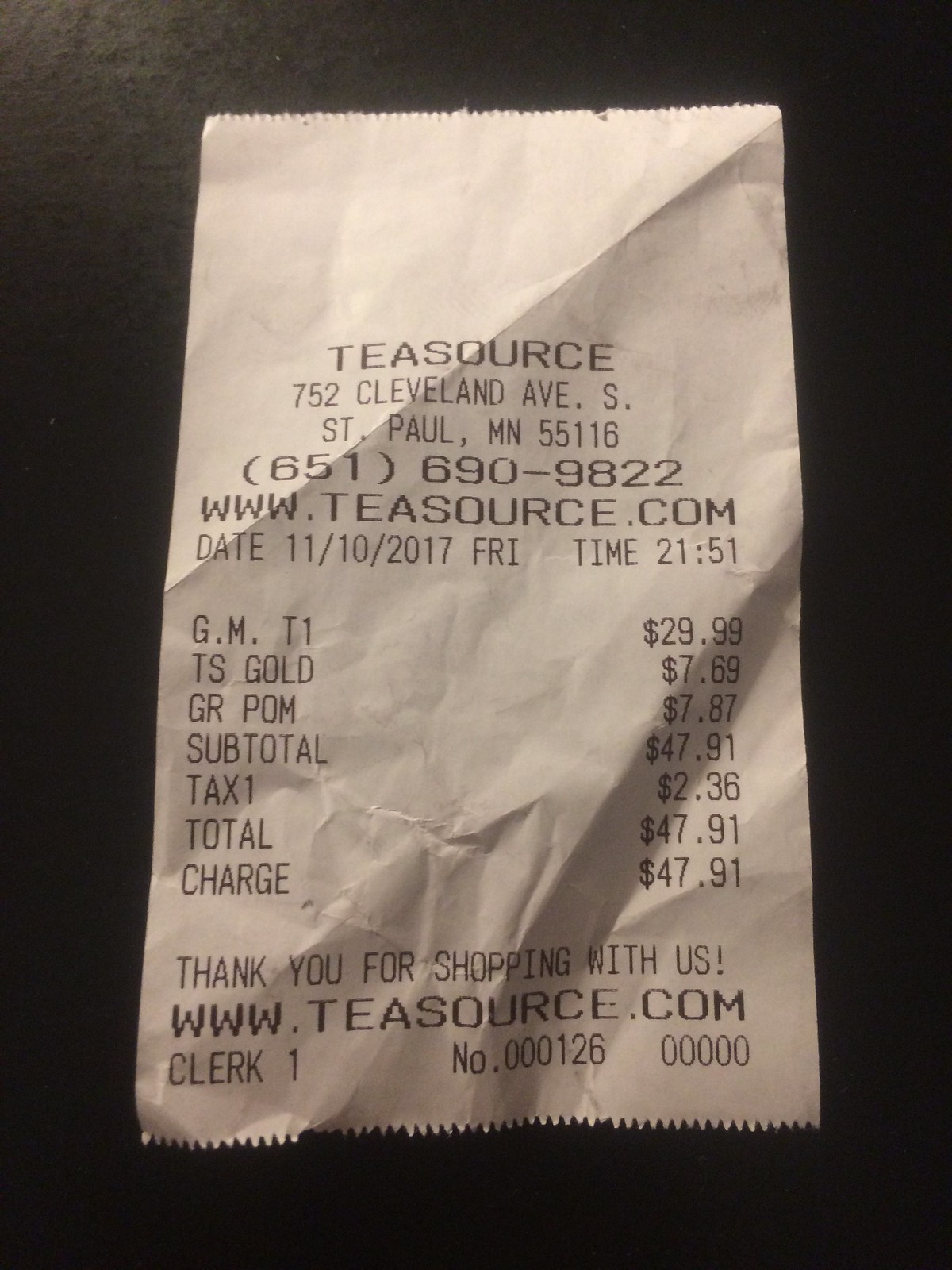This photograph showcases a well-worn receipt from T Source, a store situated at 752 Cleveland Avenue, St. Paul, Minnesota, 55116. The receipt lists the store’s contact information, including their phone number, (651) 690-9822, and website, www.tsource.com. Dated November 10, 2017, a Friday, the transaction was completed at 21:51 (9:51 PM).

The receipt provides a detailed list of various items purchased, culminating in a total of $47.91. Below the itemization, a message expresses gratitude to the customer with a note: "Thank you for shopping with us," and reiterates the store’s website. Additionally, the receipt indicates its unique identification number.

The receipt itself is white, showing signs of having been crumpled and is now creased in several places. It rests against a stark black background, highlighting its textures and details clearly.